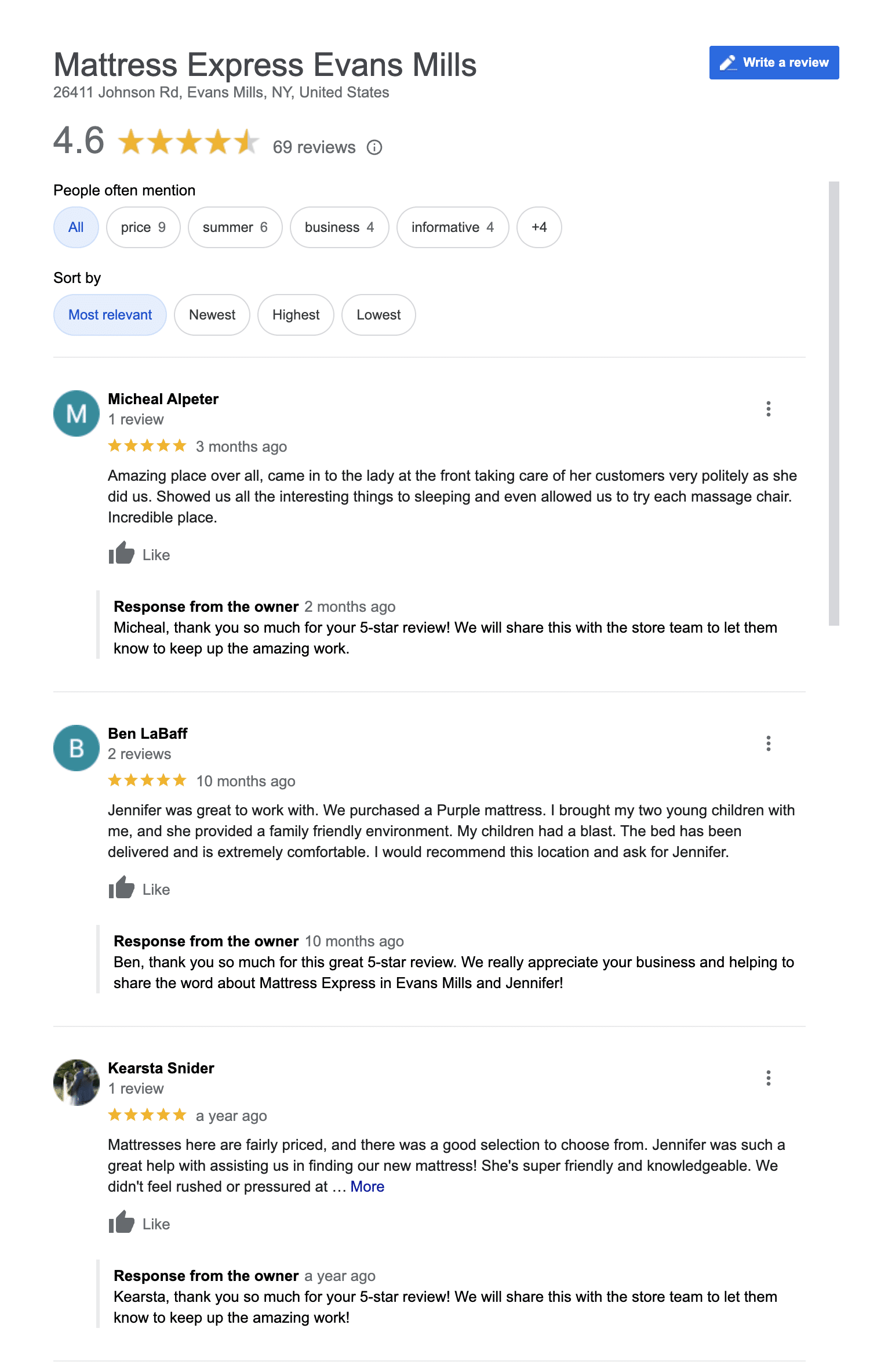The image features a review section for Mattress Express Evans Mills. 

- **Upper Left Corner**:
  - "Mattress Express Evans Mills" is written prominently in black text.
  - Below this, inside a blue text box: there is a white pencil icon.
  - The text "Write a Review" is also displayed in white within the blue box.

- **Ratings**: 
  - Directly beneath "Mattress Express Evans Mills," the overall rating is shown as 4.6 with four and a half out of five stars filled in orange.
  - The total number of reviews is mentioned as 69.

- **Common Mentions**: 
  - "People often mention" section is listed, featuring words circled in blue such as "all," "price," "business," and "information."

- **Sort Options**:
  - Below the mentions, sorting options are available with "Sort by" text followed by a blue circle indicating "Most relevant."

- **Reviews**: 
  - The first review shows an "M" inside a teal circle, next to the username.
    - This user rated the store five stars in orange, three months ago, and shared their review.
  
  - The second review has a "B" inside a green circle.
    - This review also shows a five out of five stars rating.
  
  - The third reviewer’s icon appears as a small image of a person in a white dress. 
    - Their username is listed next to the icon.
    - They provided a five-star rating in yellow, one year ago.